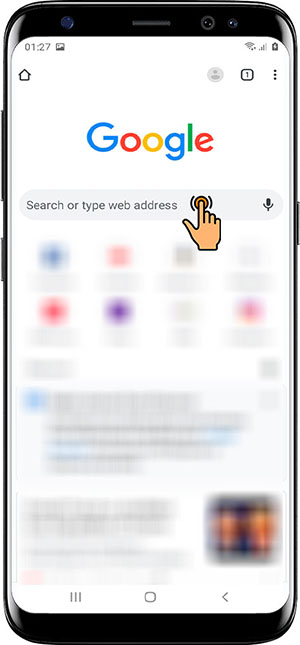A smartphone screen is displayed in the image. The phone features a distinctive design with black sections at the top and bottom, and a white rectangular body with curved corners. The screen shows the time "01:27" at the top, along with several status icons: a small image thumbnail, a Wi-Fi symbol, a signal strength indicator with lines increasing in size from left to right, and a battery icon.

Beneath these icons, there is a row of additional icons: a house symbol, a person icon, an outlined square with the number "1" inside, and a vertical trio of dots representing a menu. Following this, the word "Google" is prominently displayed in its signature colorful font, with letters in blue, red, yellow, blue, green, and red.

Below "Google," a light gray search bar is present, displaying "Search or type web address" along with icons of a hand pressing a button and a microphone for voice input.

The lower portion of the screen is heavily blurred, obscuring specific details. Despite the blur, it is evident that there are two rows of symbols accompanied by text, though the text is unreadable. A recognizable blue symbol and some additional text appear lower on the screen, with all elements dulled to a grayscale. In the lower right-hand corner, a blurred image can be seen.

Overall, this picture showcases the interface of a smartphone with a blend of clear and indistinct elements, emphasizing the Google search bar and various icons while the majority of the content remains intentionally out of focus.